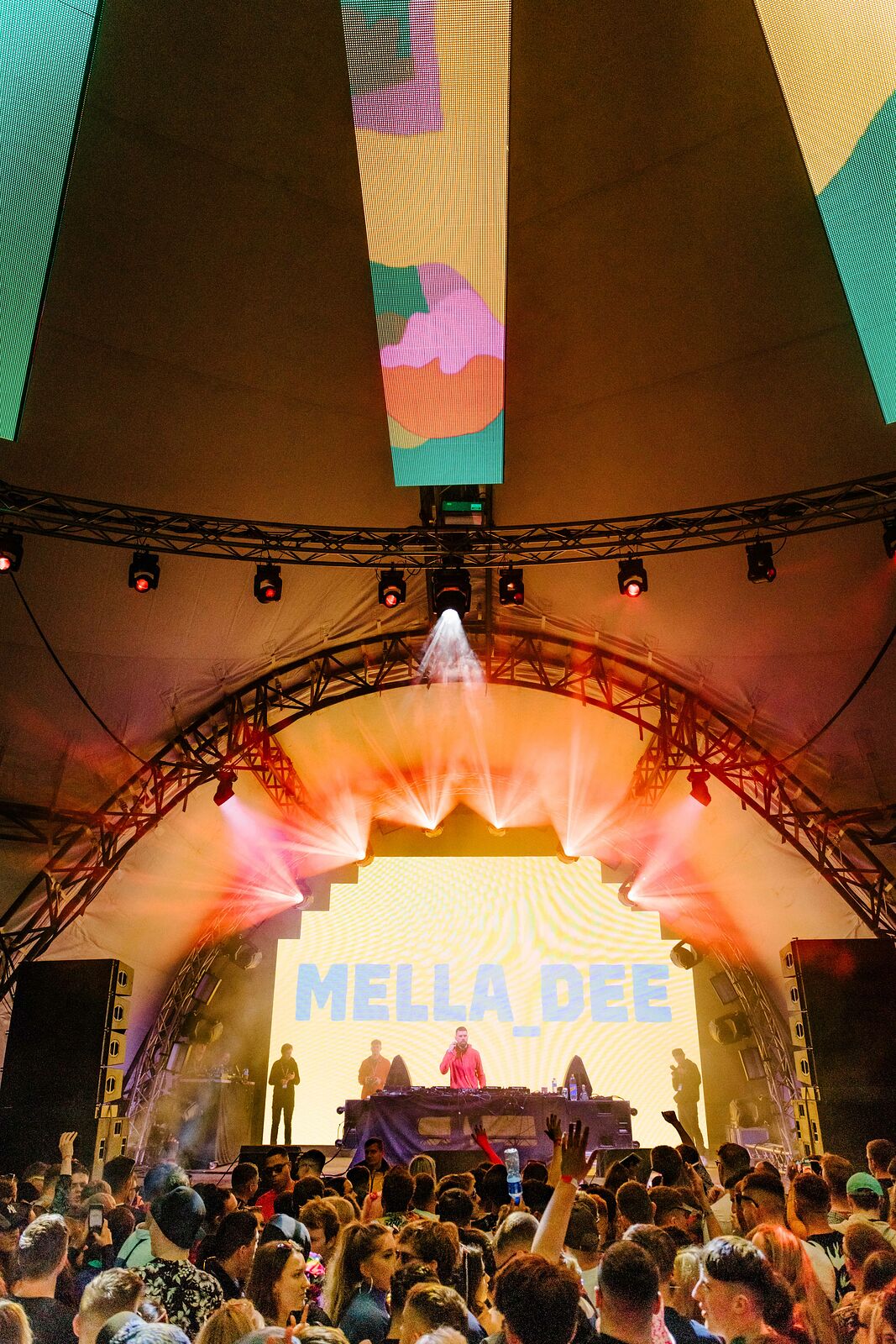This image captures a bustling concert or performance venue, distinguished by a large, semi-circular stage that forms the focal point. The stage features a curved metal girder surrounding it and is dominated by a large, bright LED screen displaying the name "Mela Di" in glowing yellow text. In front of the screen, a desk stretches across the stage, equipped with several bottles of water, resembling a DJ booth adorned with various equipment. Several individuals, indistinct in their features but seemingly young men and women, occupy the stage area. Overhead, the venue boasts a high, tent-like ceiling with metal beams and cloth resembling curtains draped across, contributing to a halo effect created by brightly shining spotlights. Additional panels in vibrant colors—purple, yellow, teal, and dark salmon red—decorate the peak of the structure, adding an abstract artistic element. The foreground reveals a large audience, some with their hands raised and others engaged in conversation, creating a vivid, dynamic atmosphere beneath the enveloping, domed ceiling.